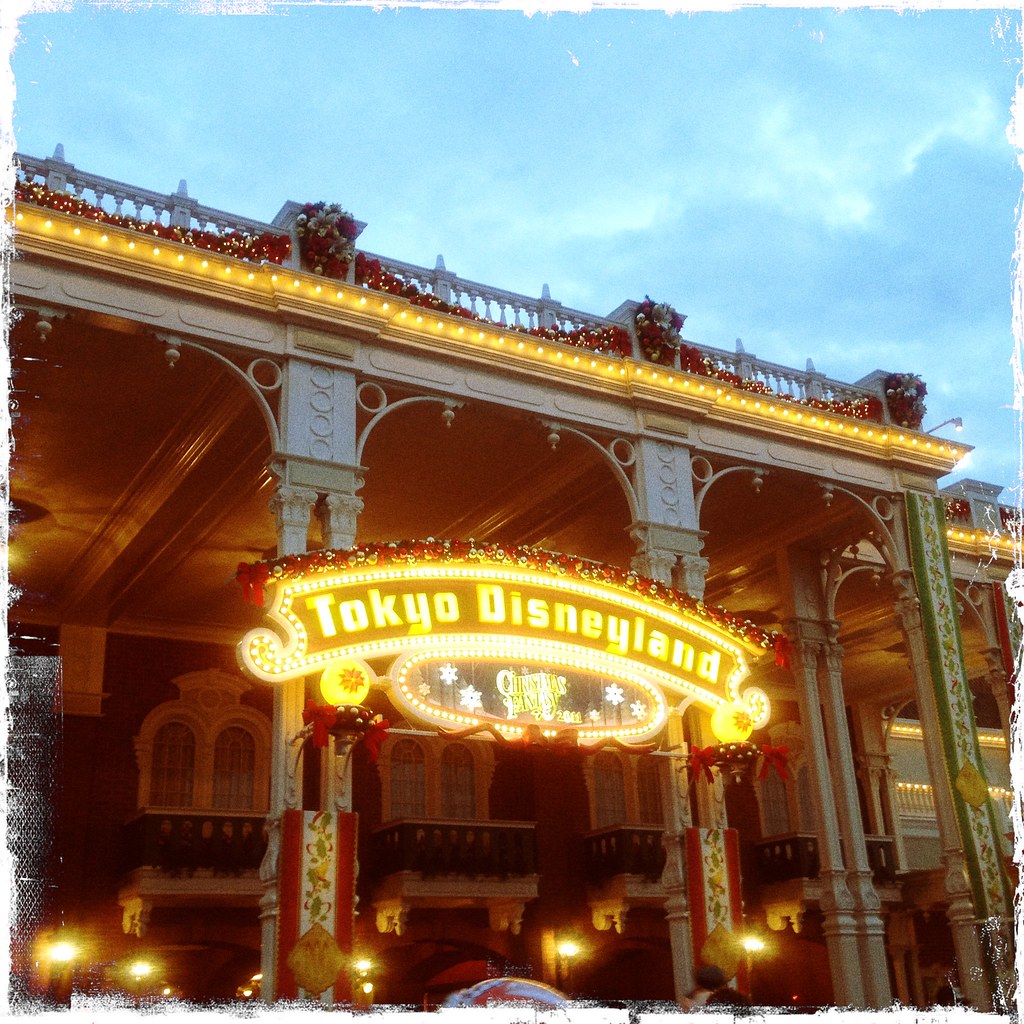This image captures the grand entrance to Tokyo Disneyland, framed by an overcast, cloudy sky. Dominating the scene is a large, bright yellow sign proclaiming "Tokyo Disneyland," adorned with festive red decorations, including gold Christmas balls with red ribbons. Beneath this sign, the words "Christmas Fantasy" are illuminated, hinting at a seasonal celebration. The building, characterized by its classic architecture featuring large columns and arched windows, is lavishly decorated with Christmas lights and various red and green embellishments. A balcony on the upper part of the structure is festooned with red and white flowers and red tinsel, enhancing the holiday atmosphere. Despite the festive setting, only a few heads of people are visible, seemingly entering the building, while the worn edges of the photograph add a nostalgic touch, suggesting it might be an old or well-loved image.